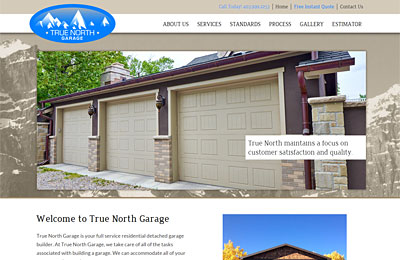"Welcome to True North Garage! This image captures the essence of our comprehensive garage-building services, emphasizing our dedication to customer satisfaction and quality craftsmanship. The main photo features a full-service, residential, detached 3-car garage. Each of the three tan garage doors is beautifully framed by pillars, with the lower half adorned in classic brick and the upper half in rich brown-painted wood panels. Surrounding the garage, a serene setting is depicted with a clear blue sky and striking yellow trees, adding a touch of natural beauty. At True North Garage, we manage every aspect of the garage construction process, ensuring that we can meet all your needs efficiently and to the highest standards."